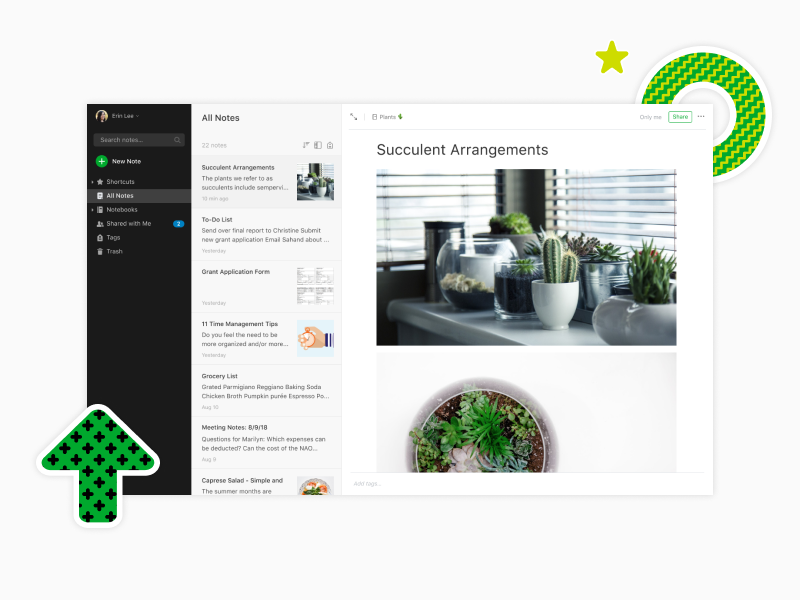The horizontally rectangular image features a light gray background and showcases a screenshot, likely from a blog, website, or social media platform. The left side of the frame has a vertical black banner with a list of options, among which "All Notes" is highlighted. Although the text is somewhat small and difficult to read, other options are listed below. Adjacent to the banner, a vertically rectangular section also on a light gray background displays the heading "All Notes" at the top, followed by a neatly arranged list: "Succulent Arrangements," "To-Do List," "Great Application Form," "11 Time Management Tips," "Grocery List," "Meeting Notes," and "Caprice Salad." Occupying a little more than half of the horizontal space, the remainder of the frame highlights the heading "Succulent Arrangements" and features two images displaying various succulent plants.